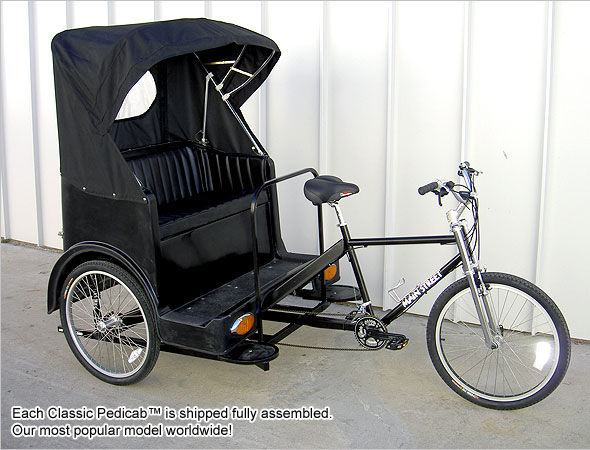The image showcases a black tricycle-style vehicle with a pedal and a seat compartment, commonly known as a pedicab. The pedicab, which is facing slightly to the right, features a small black buggy, integrated as part of the vehicle, with its back wheels serving as the tricycle's rear support. The buggy has a top covering and a plastic window at the back. Additionally, there are two amber-colored lights located at its base.

The tricycle is set against a white-colored wall and rests on a gray surface, likely cement. The right side of the vehicle is primarily visible. A white marking can be seen on the bar ascending from the gears to the front, although it is unclear what it says.

Text on the image, located in the bottom left corner, reads, "Each classic pedicab is shipped fully assembled. Our most popular model worldwide!" The lettering is in black with a white outline.